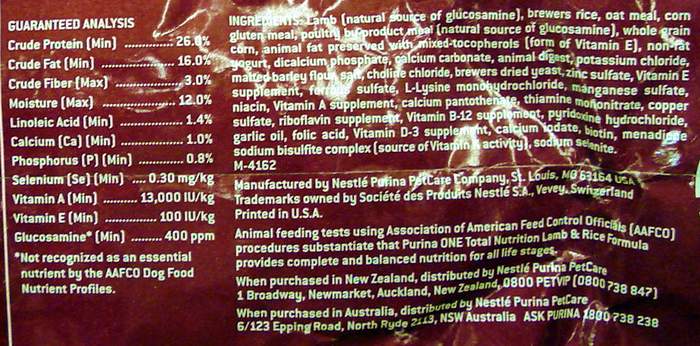This image shows the ingredients label on the back of a bag of pet food. The background of the label is a reddish brown color, with all text displayed in white font. The left-hand side of the image features a "Guaranteed Analysis" section. This section includes a detailed percentage breakdown of key nutritional components such as crude protein, crude fat, crude fiber, moisture, and several vitamins.

On the right-hand side, the ingredients are listed in descending order of predominance. The first ingredient is lamb, followed by brewers rice, oatmeal, corn, gluten meal, and poultry by-product, among others. Below the list of ingredients, there is a paragraph providing information about the manufacturer, Nestle Purina Pet Care Company. This section also includes details about animal feeding tests and relevant addresses for further contact.